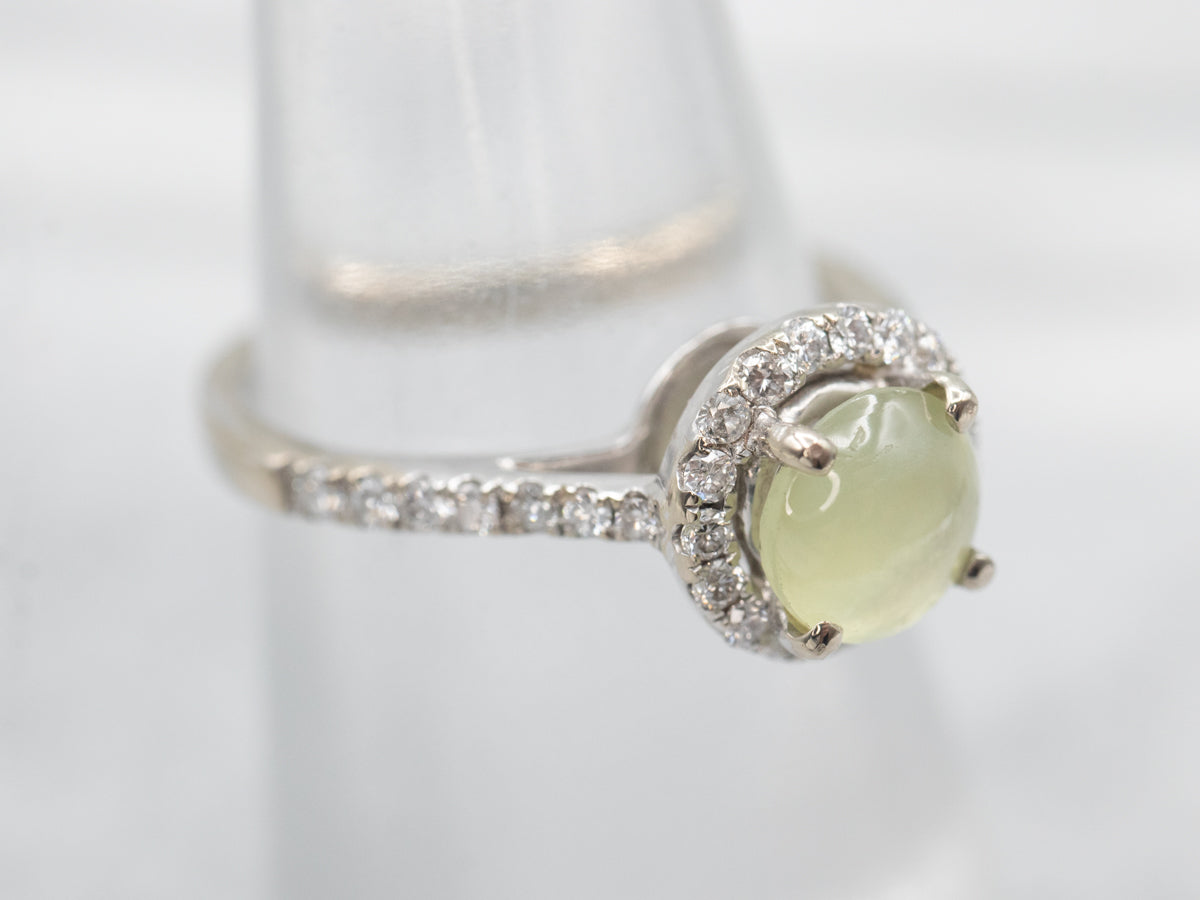The image showcases a sophisticated diamond ring displayed on a clear ring stand, likely in a jewelry store setting. The ring features a round, flat central gemstone with a light yellow or yellow-green hue, held securely by four prongs. This elegant stone is surrounded by smaller channel-set diamonds that form a striking halo. The band, crafted from either white gold or platinum, also boasts channel-set diamonds, which extend halfway around. The individually embedded diamonds on both the band and the setting add a layer of intricate sparkle, making this piece exceptionally captivating and likely very valuable. The close-up shot reveals the meticulous details and craftsmanship of the ring, emphasizing its luxurious allure.